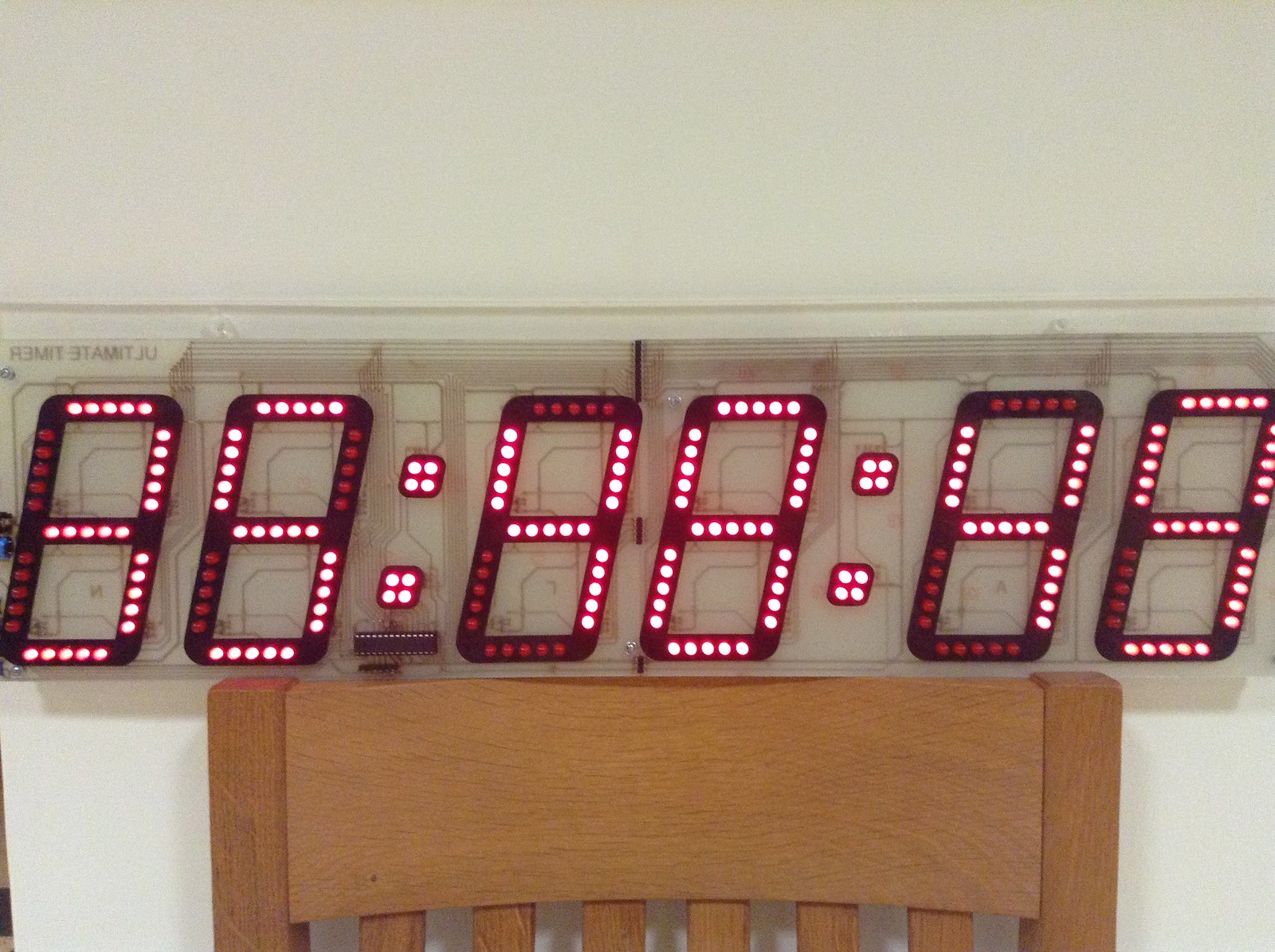This image depicts the interior of a home with a white-painted wall and the upper portion of a light brown wooden dining chair positioned against it. Mounted slightly above the chair is a rectangular digital clock, labeled as "Ultimate Timer." The clock is large and features a light brown and gray design with distinct lines and shapes in its background. The main display of the clock consists of six sections with LED circles emitting red light. These circles form the numbers 35:48:49, with dots separating the groups. The exact meaning of these numbers is unclear, but they might represent hours, minutes, and seconds. The visual setup suggests the clock is mounted relatively low on the wall, possibly at chair height.